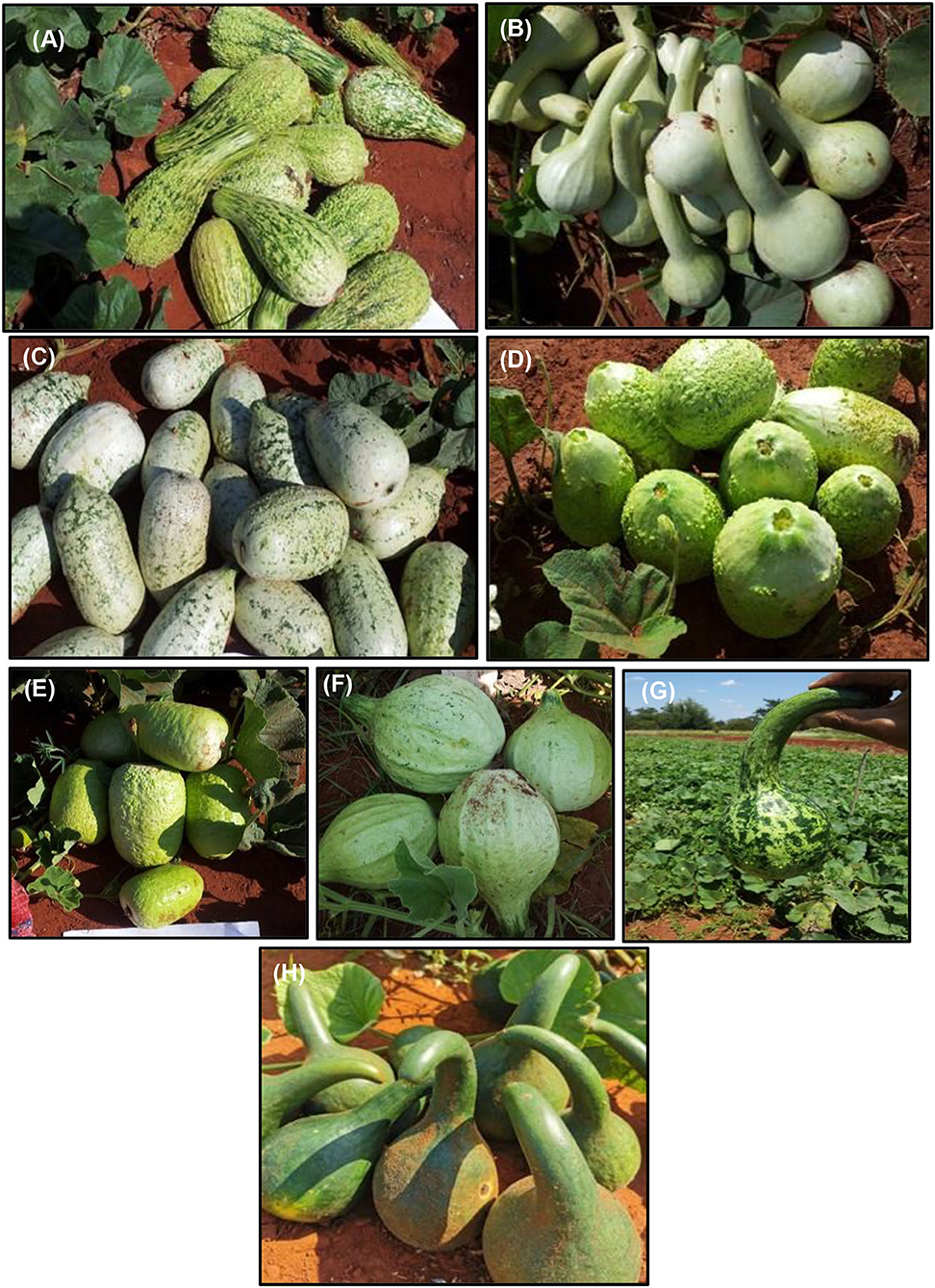The image is a detailed collage of eight labeled photographs (A through H) showcasing various types of organic produce, primarily gourds and fruits, placed on a dirt background with some leaves scattered around. The photographs are separated by thin white lines. The top left picture (A) features gourds on a brown table, while the one directly below it (B) shows whitish gourds with tubular protrusions. Picture C, in the next row, displays lighter green gourds resembling jelly beans, and picture D shows darker green gourds, also jelly bean-shaped. Pictures E, F, and G continue the theme of various gourds and squash in different shades of green. The bottom center photograph (H) highlights more mature gourds, green in color, with rounded bases and long handles. The collage captures both indoor and outdoor settings, emphasizing the diversity and natural beauty of the produce.